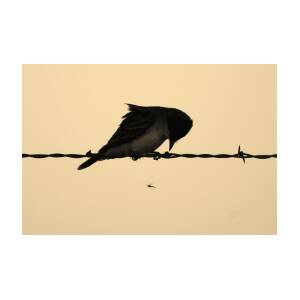The image features a small photograph with an off-white, beige background. Dominating the scene is a dark silhouette of a bird perched on horizontally stretched barbed wire, positioned centrally. The bird, with short, black feathers, is seen roosting quietly, its tail extending to the left side of the picture. Its head is bowed downwards, beak almost touching the wire as if pecking at something unseen. The barbed wire is intricately coiled, framing the bird in stark, shadowy relief. Underneath the wire, there is a noticeable black smudge whose origin is ambiguous, adding to the photograph's minimalist yet striking composition.